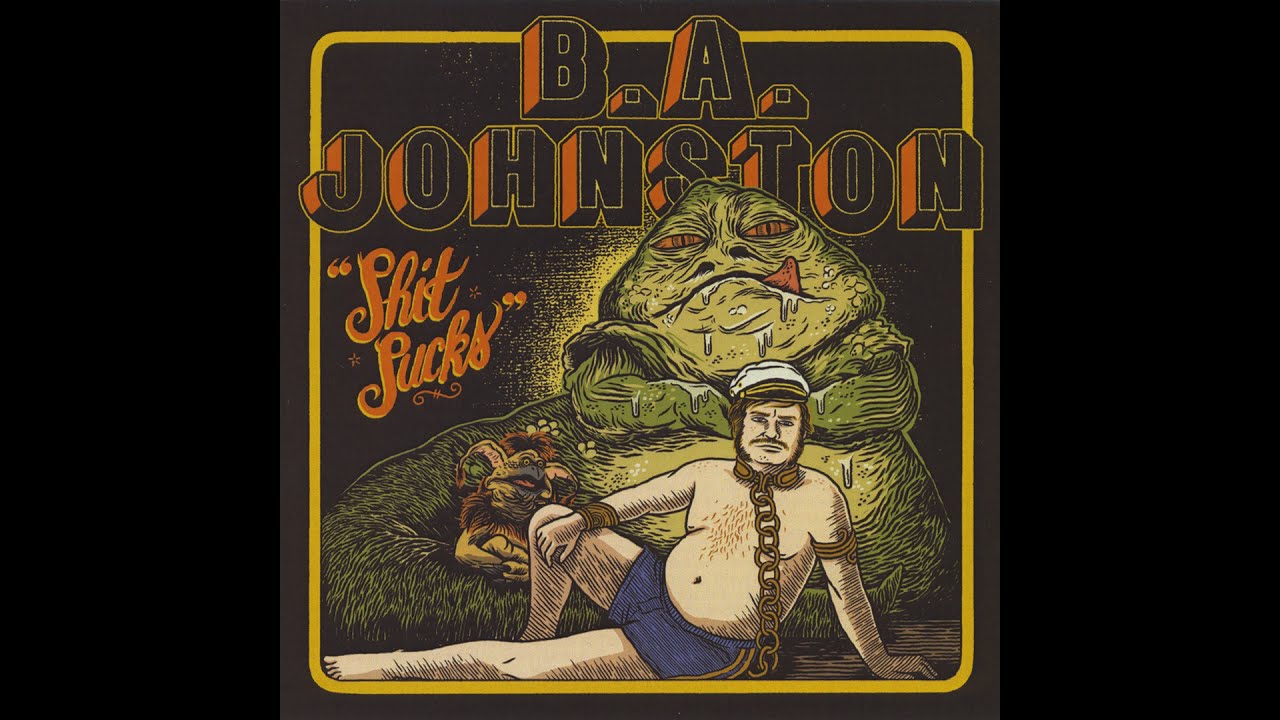The image resembles an old cartoonish album cover with heavy Star Wars influences. It features a black background with a yellow stripe around the edges, creating a border for the central elements. At the top, bold red and black letters spell out "B.A. Johnston," while a quote in the middle-left reads "SHIT SUCKS" in a distinct, spaced-out format.

The central illustration prominently includes a green, slobbering Jabba the Hutt with his tongue sticking out and red eyes. In front of Jabba, a chubby man with a white captain's hat, reminiscent of a skipper's hat from Gilligan's Island, is depicted leaning on the ground. He is shirtless, wearing blue swim trunks, and has a chain around his neck that drapes forward and behind him. The man's pose has one hand resting on the ground, the other on his bent knee. Jabba's imposing figure looms behind this individual, reinforcing the Star Wars theme.